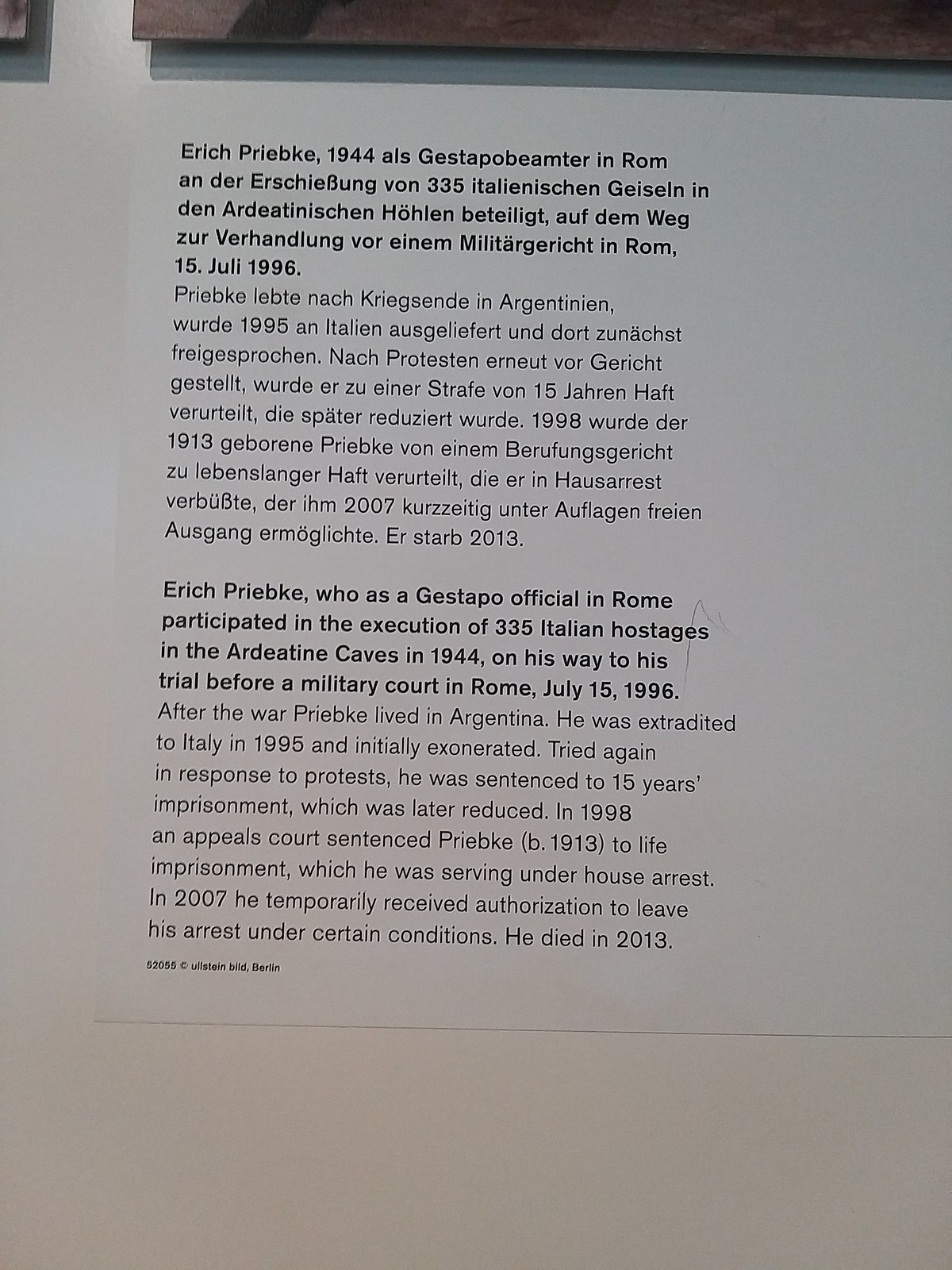The image depicts a white piece of paper or card affixed to a surface, possibly a wall, and slightly below a picture frame. The top portion of the text is in German, while the bottom half offers an English translation. The text details the biography of Eric Priebke, a Gestapo official in Rome who participated in the execution of 335 Italian hostages in the Ardeatine Caves in 1944. The narrative continues, stating that Priebke was extradited from Argentina to Italy in 1995, initially exonerated, but later retried due to public protests and sentenced to 15 years imprisonment, later reduced. In 1998, an appeals court sentenced him to life imprisonment, which he served under house arrest. The text also notes that in 2007, Priebke temporarily received authorization to leave under certain conditions. He died in 2013.